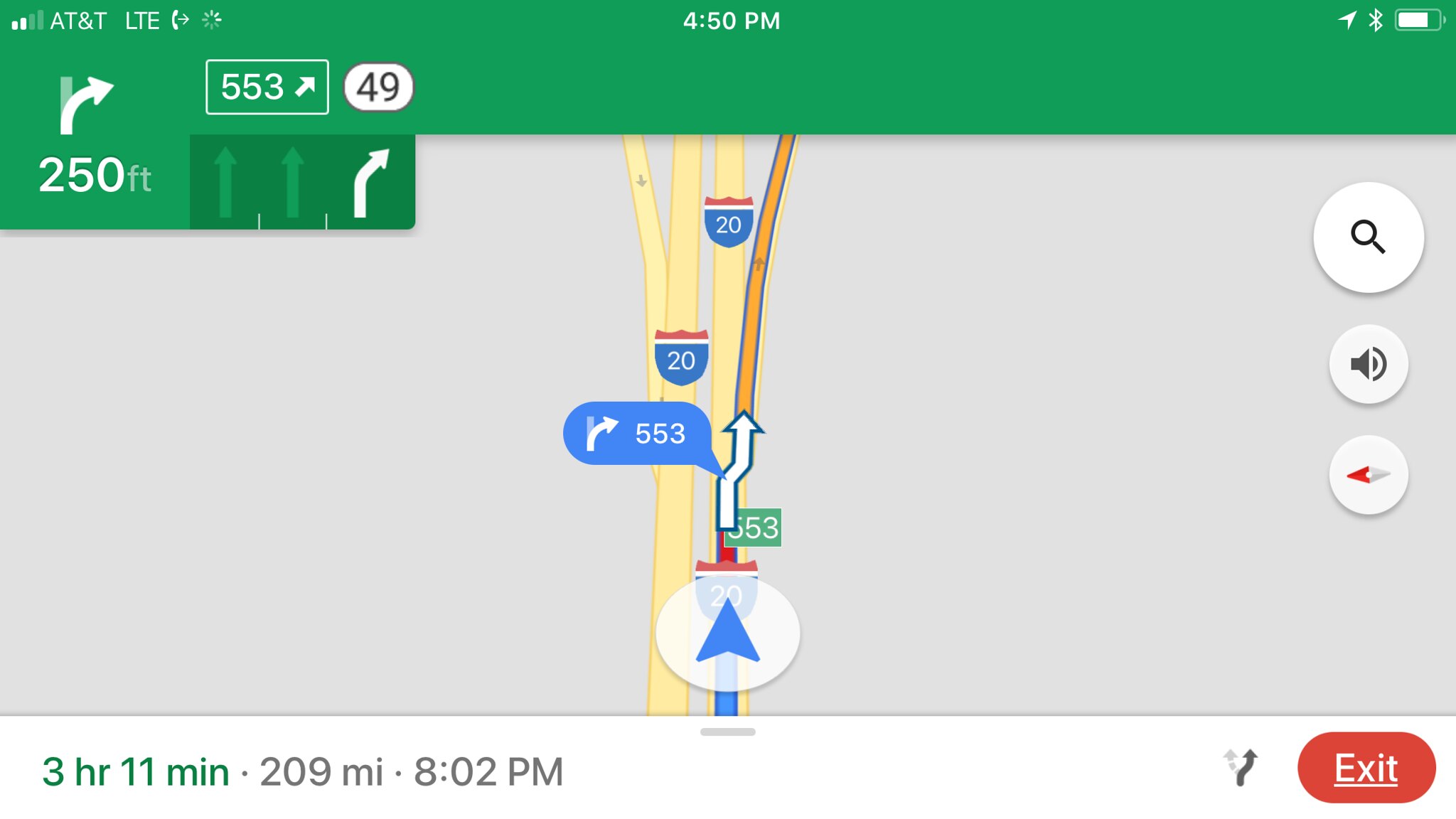This image is a screenshot from a smartphone displaying Google Maps in landscape orientation, captured at 4:50 PM. The service provider is AT&T with LTE connectivity, showing two bars of signal strength, and the battery level is approximately 80%. Bluetooth is enabled. 

In the upper part of the screen, a green bar indicates an active navigational route. The user is instructed to take Exit 553 on Route 49, located 250 feet ahead to the right. The route details present multiple directional arrows with green and white signage, indicating how to merge and exit. On the left side, there are icons for search, sound, and navigation options.

The map itself shows the primary thoroughfare, Interstate 20, in yellow, with the upcoming exit highlighted in orange. The route guidance at the bottom states that the journey will cover 209 miles, taking approximately 3 hours and 11 minutes, with an estimated arrival time of 8:02 PM. The current vehicle location is indicated by a moving blue arrow within a circle.